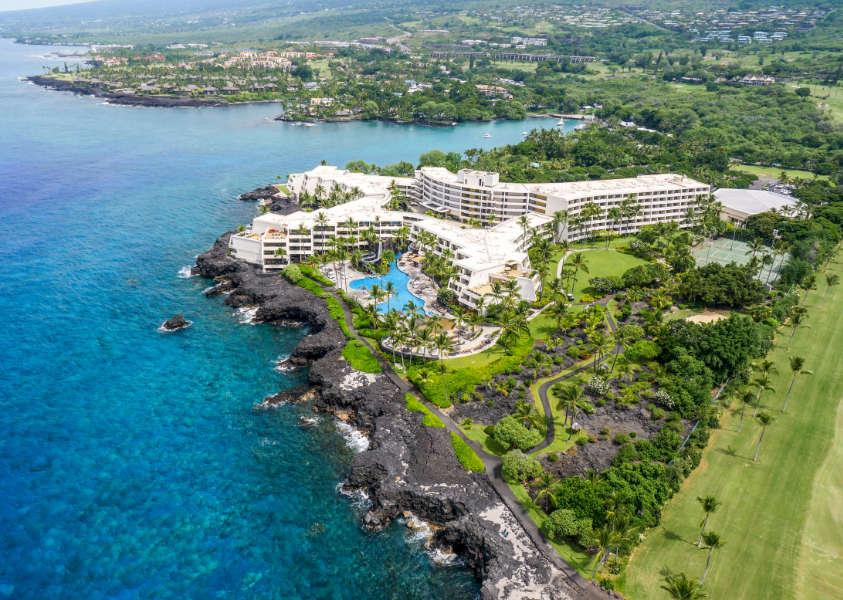This aerial image captures an expansive resort complex shaped like an X, or with four prongs, situated on a rugged, rocky coastline. The central focus is the large, flat-roofed, white main building, which is likely a hotel or country club. In front of the building lies a large, wavy-shaped pool that sits between the hotel and the striking cerulean blue ocean. The coastline directly in front of the resort features dramatic black lava rocks, devoid of a sandy beach.

To the right of the resort, a tennis court is partially visible, and farther to the right, there appears to be a grassy area that might be part of a golf course. The image also shows the road leading up to the resort, surrounded by lush trees and green spaces. In the upper right corner, a distant town is faintly visible in another bay. Scattered boats and houses can be seen further back from the rocky shoreline, contributing to the vibrant, multifaceted landscape captured in this stunning aerial shot, which appears to have been taken by a drone.